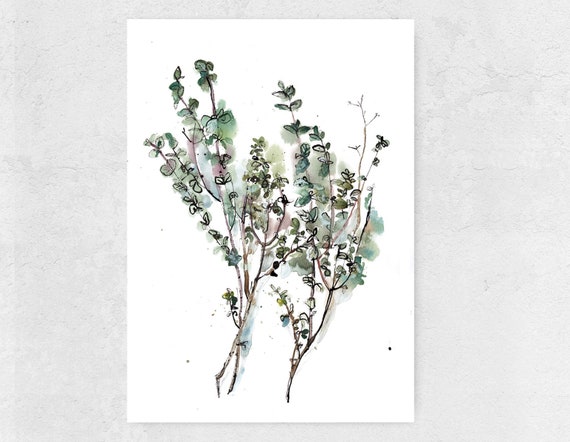The image depicts a rectangular white canvas centered against a blotchy light gray background that resembles a spackled concrete wall. The canvas showcases a delicate watercolor painting of three spindly, thin light brown branches. The branches, positioned with two crisscrossing on the left and another separate branch to the right, taper upward with numerous small twigs. Adorning the branches are round leaves painted in shades of green and some with hints of blue. The background of the canvas features splashes of light green paint, adding depth and texture to the soft, artistic composition.